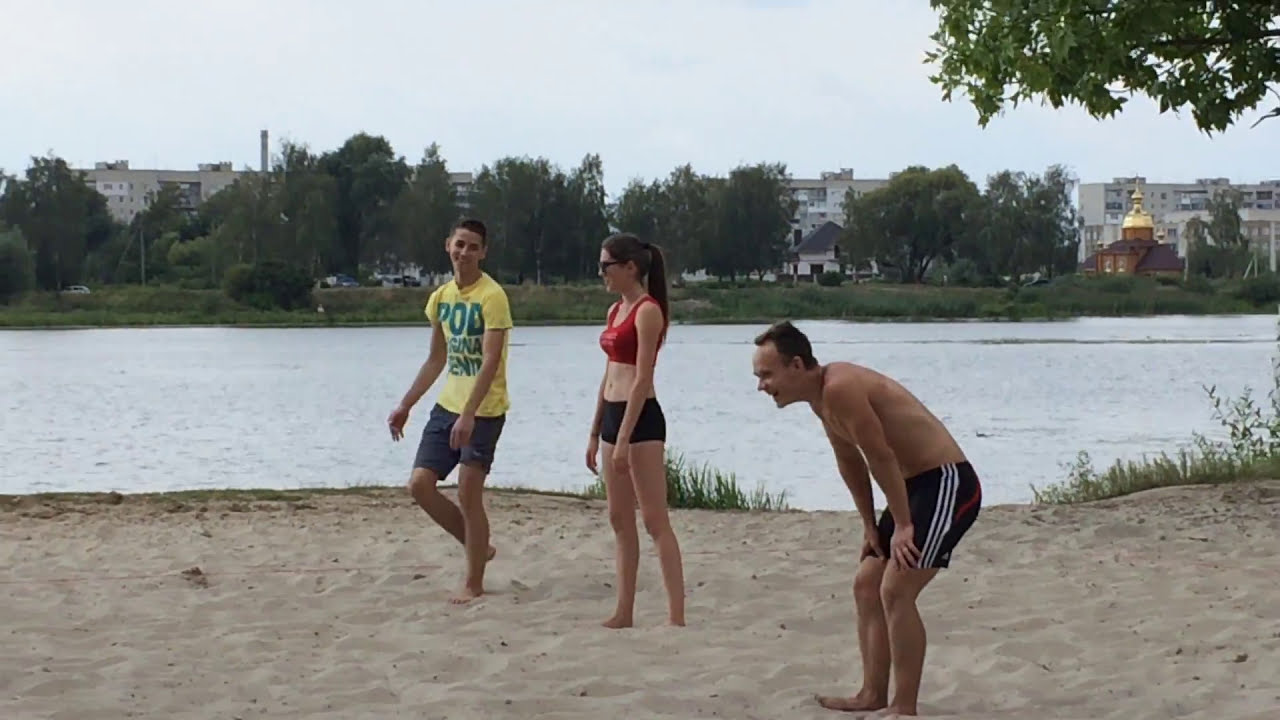The photograph captures a scenic view of a sandy beach bordering a lake, with three people in the foreground. To the left stands a young man with brown hair and a tan complexion, dressed in a yellow shirt with green lettering that reads "P.O.D.", paired with blue shorts. Directly to his right is a woman with long black hair tied back into a ponytail, sporting a red bikini top and black boy shorts. She also wears black sunglasses and appears to be in her 20s. On the far right, a shirtless man with short brown hair and a white complexion is hunched over with his hands on his knees, wearing navy blue shorts adorned with three white stripes. The lake in the background has a light grayish-blue tint and gentle ripples, extending towards a distant shoreline lined with green grass and dense trees. Beyond the trees, several multi-story buildings with gray and brown façades rise against a hazy, overcast sky, with a notable structure featuring a golden dome peeking through the foliage. The entire scene is bathed in a muted light, adding a serene quality to the overall composition.